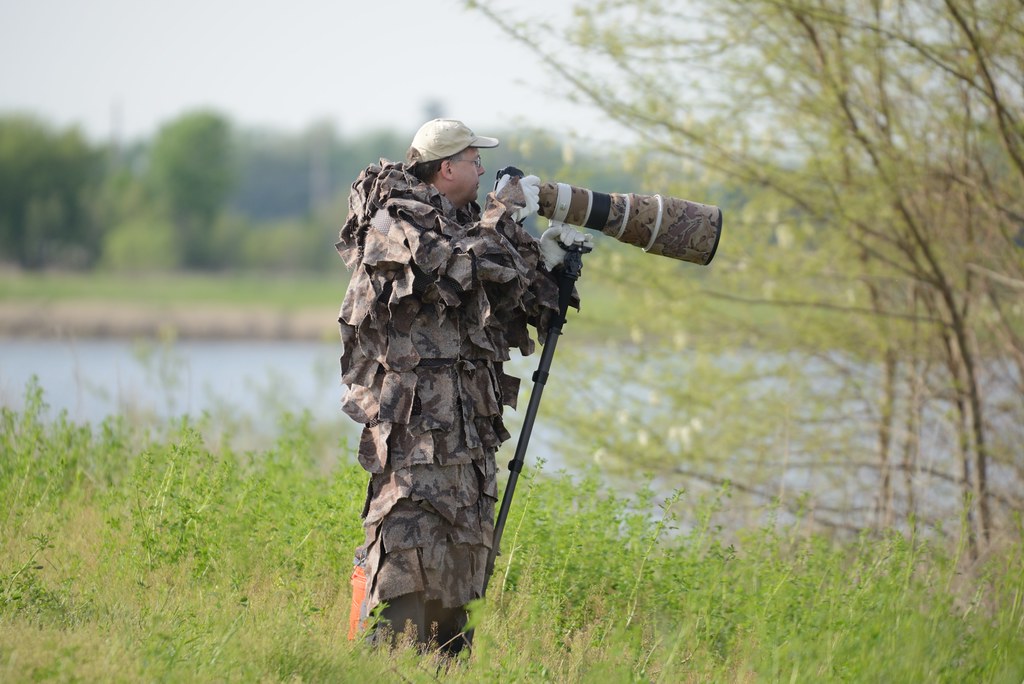In this detailed photograph, a photographer is standing amidst knee-high tall grasses by the edge of a body of water, which appears to be a lake or a river. The background of the image is slightly blurred but reveals some buildings, trees, and the expanse of the water. The photographer is dressed in an elaborate camouflage outfit, consisting of numerous separate pieces sewn or tied onto the outer layer of his clothing to mimic the appearance of leaves and natural surroundings. He is wearing a light beige or white baseball cap, and white glasses are discernible on his face. In his hands, he holds a camera with a very long lens, covered in plastic for protection, which is mounted on a tripod. The photographer is intently aiming his camera towards the lake, capturing the scene beyond.